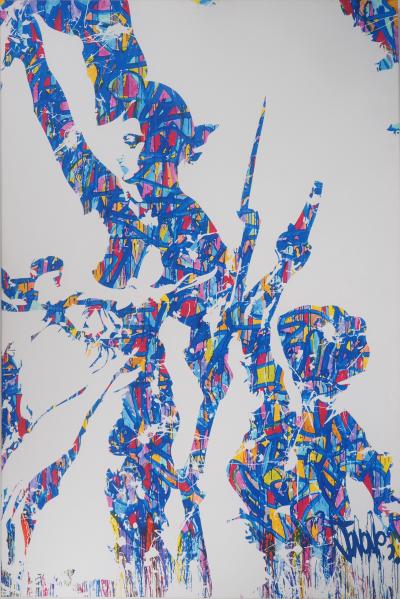The image is an abstract painting featuring two indistinct human figures set against a predominantly white background. The figures, possibly women, are constructed using vibrant, mixed colors including blue, yellow, red, and orange. The colors form squiggly and blocky shapes, with blue often acting as an outline for the other hues. The person on the right, located in the lower half, appears to be facing left with something in their right hand and their left hand positioned behind them. The other person on the left side seems to be raising their right arm, possibly holding a gun, creating a dynamic clash between the two figures with a lightning bolt-like shape in the middle. Both figures are rendered in a stylized, collage-like manner, giving the impression of a rebellion or battle scene. The bottom right of the painting features what looks to be a signature, possibly reading "Jade."